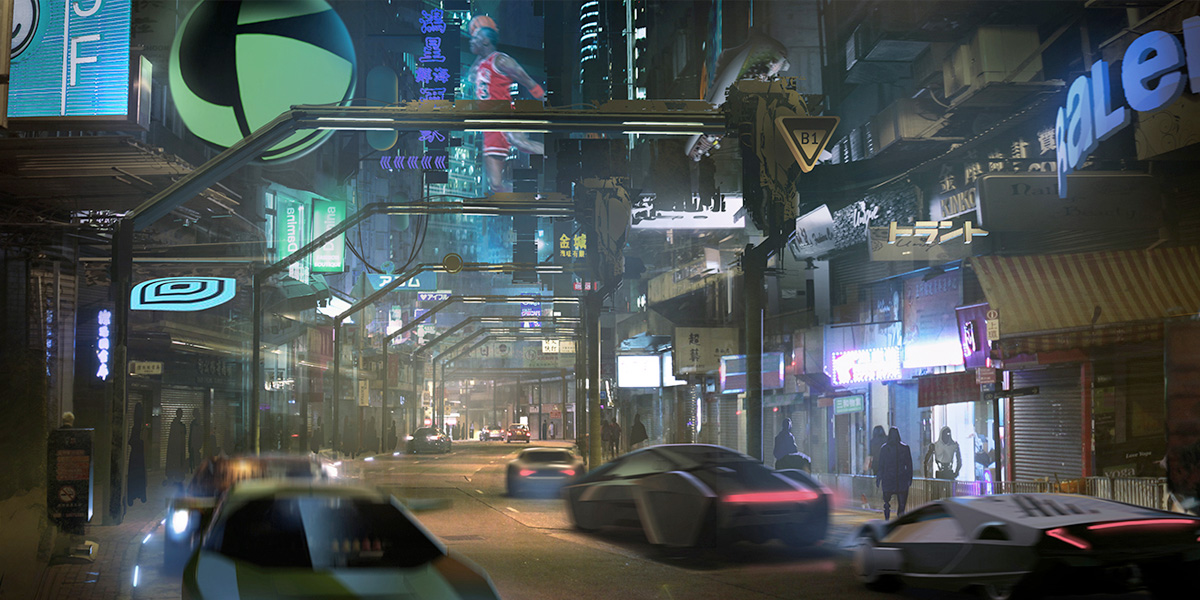In this highly stylized, cyberpunk-inspired night scene, we observe a bustling city street that exudes a cinematic quality reminiscent of Blade Runner or Ghost in the Shell. The environment is characterized by its dark, atmospheric lighting, punctuated by vibrant neon lights from storefronts and large, colorful signs. The street is populated with sleek, modern concept cars featuring distinctive red panels across their rears, driving along two lanes of traffic that bend to the right at the bottom of the image.

Pedestrians navigate the sidewalks amidst small shops adorned with neon signs displaying both Japanese and English text. The cityscape is dominated by towering buildings and metal rafters crisscrossing overhead, lending a futuristic feel. Among the visual highlights is a striking hologram of a basketball player, several stories tall, that hovers in the center, adding to the dynamic energy of the scene. Additionally, sponsor signs and billboards featuring various texts and images, including one of a jumping basketball player in red and some in Russian and Asian scripts, further enrich the scene's intricate details. This 3D render or concept art captures the essence of a lively, futuristic metropolis teeming with activity and vivid visuals.